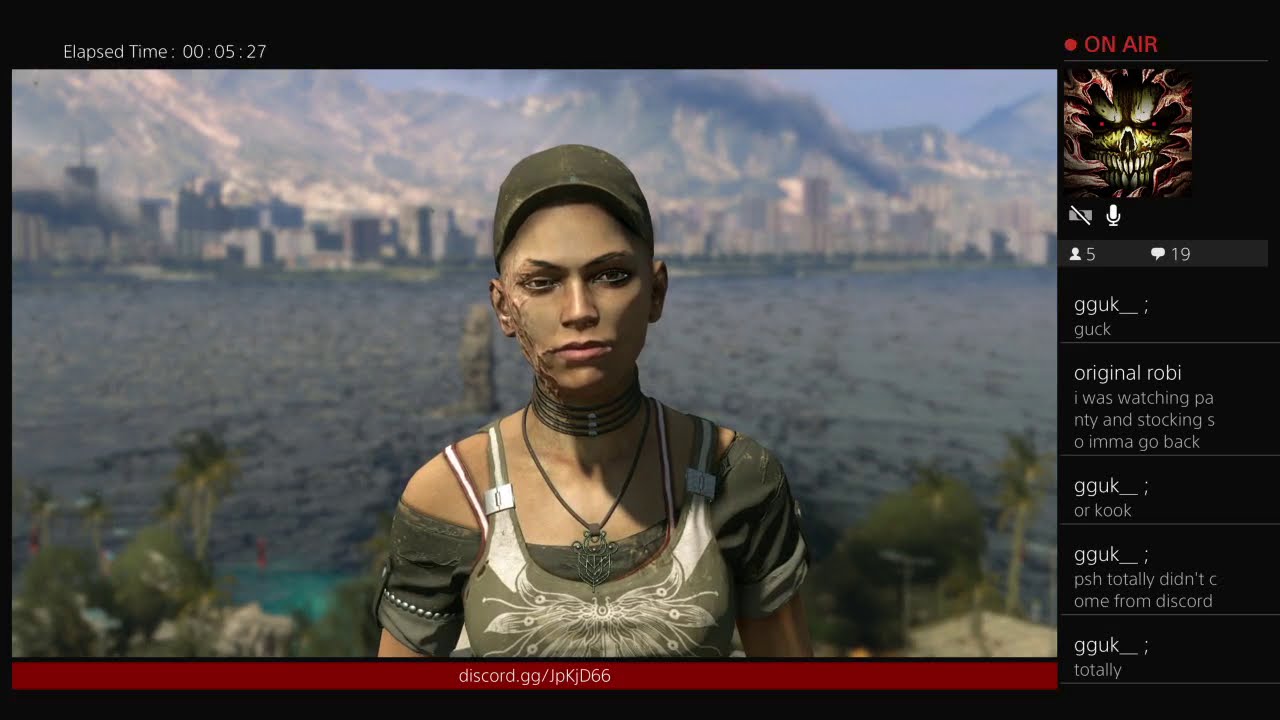The image is a detailed screenshot from a live-streamed video game, displaying a mix of visual and interface elements characteristic of a Discord gathering. Dominating the foreground is a life-like, virtual female character wearing a layered outfit consisting of a brown tank top adorned with a winged creature design and a green off-the-shoulder shirt underneath. She is also donning an olive green cap, and her face is marred with scars, suggestive of a mutated or zombie-like transformation. In the background, a picturesque landscape unfolds featuring a blue body of water, a bustling city skyline with billowing smoke, and a verdant mountain range.

To the right side of the image, a black vertical bar displays a real-time chat where five participants have made 19 comments. Distinct messages like "Guck" and "I was watching Panty and stockings" are visible. At the top of this chat section is an avatar of a demonic skull with sharp teeth, reinforcing the game’s eerie theme. Above the main game display, a black strip reads "elapsed time 00:05:27" on the left and "on air" in red font next to a microphone icon on the right, indicating the live-stream status. A Discord link is subtly placed at the bottom edge, further emphasizing the communal aspect of the scene.